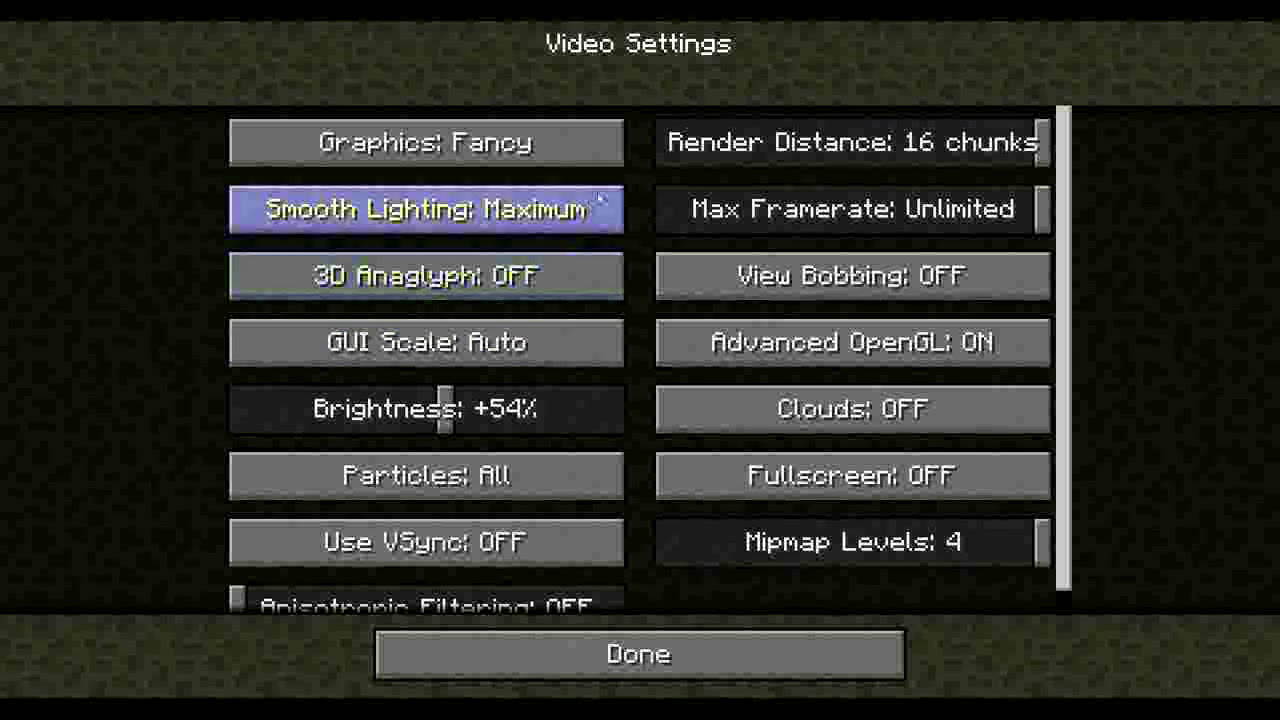The image is a rectangular screenshot of the video game Minecraft's settings menu, featuring a backdrop of a dark, low-resolution stone texture with distinct army green and gray blotches, almost resembling a leopard print. At the top center, the text "Video Settings" is prominently displayed in white. Below this, the settings are organized into two columns of rectangular boxes in varying shades of gray and purple, all centrally aligned and evenly spaced.

The left column includes settings such as:
- "Graphics: Fancy"
- "Smooth Lighting: Maximum" (highlighted in a purple box)
- "3D Anaglyph: Off"
- "GUI Scale: Auto"
- "Brightness: 54%" (with an adjustable slider)
- "Particles: All"
- "Use VSync: Off"

The right column lists:
- "Render Distance: 16 chunks" (with an adjustable slider)
- "Max Frame Rate: Unlimited" (with an adjustable slider)
- "View Bobbing: Off"
- "Advanced OpenGL: On"
- "Clouds: Off"
- "Fullscreen: Off"
- "Mipmap Levels: 4" (with an adjustable slider)

Horizontally spanning the top and bottom of the image are lighter green banners with light gray blotches, enhancing the visual segmentation of the menu. At the bottom, there is a thin gray bar featuring the word "Done" centered within it, which serves as the actionable button to exit the settings menu.